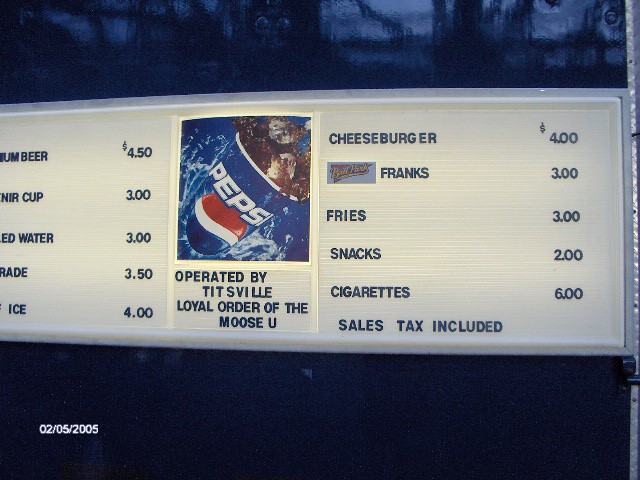This image showcases a vintage menu board with a distinct nostalgic touch, evident from its dated pricing. The board has a blue background, and at the bottom, the year "2005" is prominently displayed in white letters, suggesting its issuance date. The menu includes a variety of items and their respective prices, all written in blue letters and numbers.

The beverage section lists:
- Premium Beer: $4.50
- Souvenir Cup: $3.00
- Bottled Water: $3.00
- Gatorade: $3.50
- Ice (possibly shaved ice): $4.00

The food section reads:
- Cheeseburger: $4.00
- Ballpark Franks: $3.00
- Fries: $3.00
- Snacks: $2.00
- Cigarettes: $6.00

A notable detail is the inclusion of "sales tax included" in the prices, and the board is operated by "Titusville, loyal order of the Moose U." Additionally, there are images of a Pepsi can and a Pepsi cup filled with ice and the beverage, merging with the white and blue theme of the background.

The overall appearance and especially the low prices, compared to current standards, emphasize the menu board’s age.